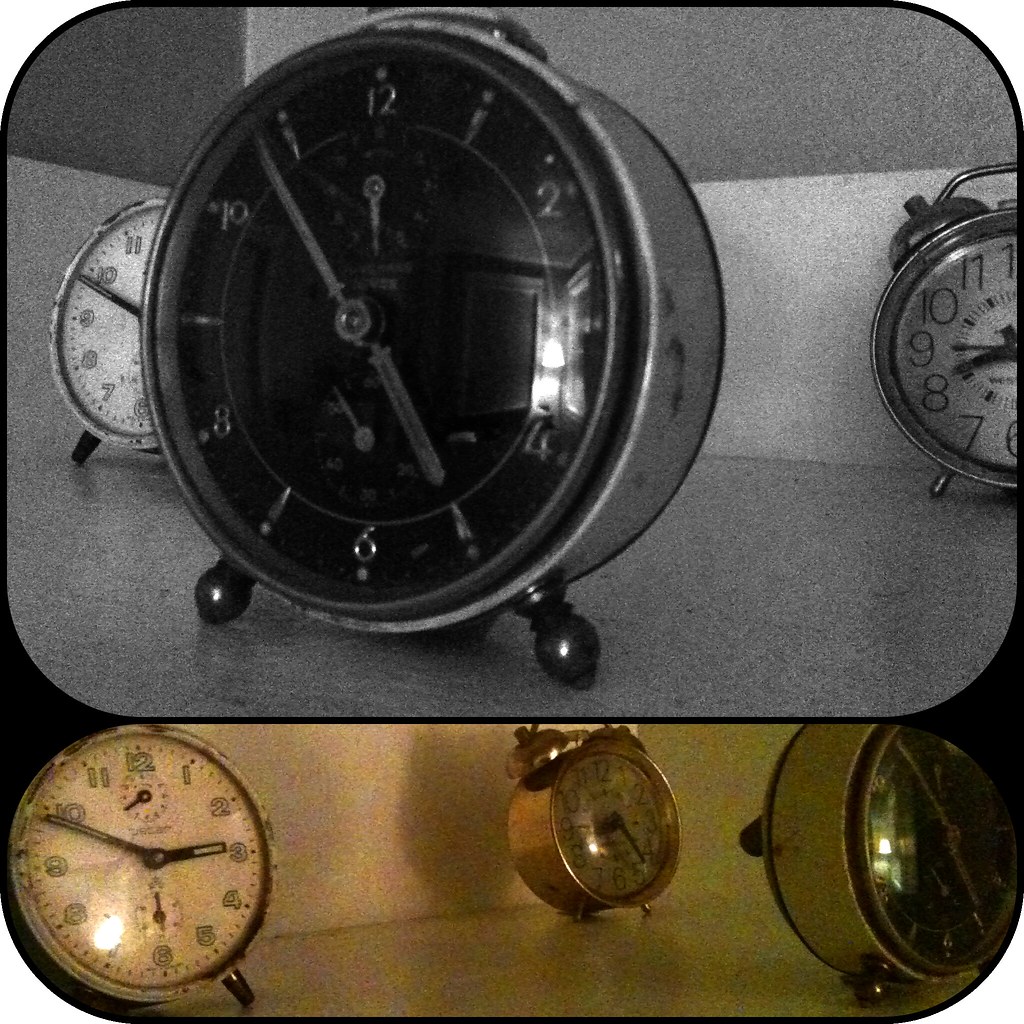This composite image features two distinct yet thematically connected photographs, vertically aligned with rounded corners encased in a thin black frame. The upper image, occupying approximately two-thirds to three-quarters of the overall space, is presented in black and white with pronounced film grain, evoking a vintage aesthetic. It showcases three old-fashioned alarm clocks placed on a table; the nearest clock is predominantly black, while the two in the background feature white faces. The lower portion of the composite, which takes up the remaining quarter of the space, transitions to color, albeit with noticeable digital noise. This section also captures the same trio of alarm clocks, albeit rearranged on the table, creating a subtle visual narrative between the two images.